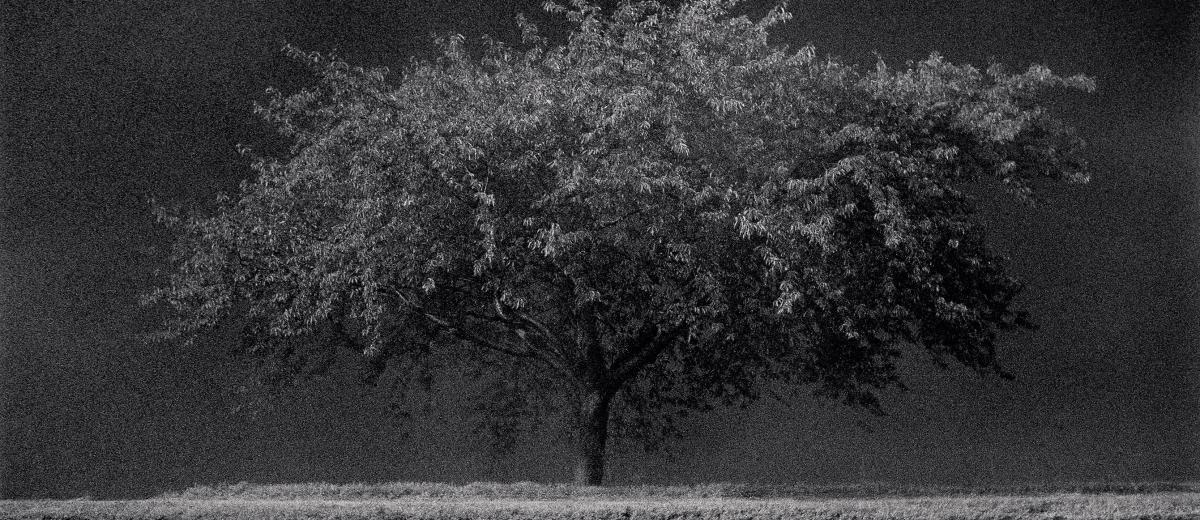This black and white image showcases a fully-grown, broad tree positioned centrally on a flat, grassy field. The tree's dramatic expanse, with branches extending widely to the left and right and leaves almost reaching down to the ground, gives it an overgrown and unkempt appearance. The dark background contrasts sharply with the lighter tones at the top of the tree, creating deep shadowing at the bottom and on the leaves. Despite the clarity of details, it remains uncertain whether it is a photograph, a digital rendering, or a hand-drawn piece, and whether the scene represents night or day. The rectangular frame is entirely dominated by the tree, leaving no other elements or text visible, lending a sense of isolation and focus on the tree's intricate details. The trunk is relatively short, giving room for the branches and leaves to spread out and fill the image, almost like a weeping willow, though the exact type of tree is indiscernible.